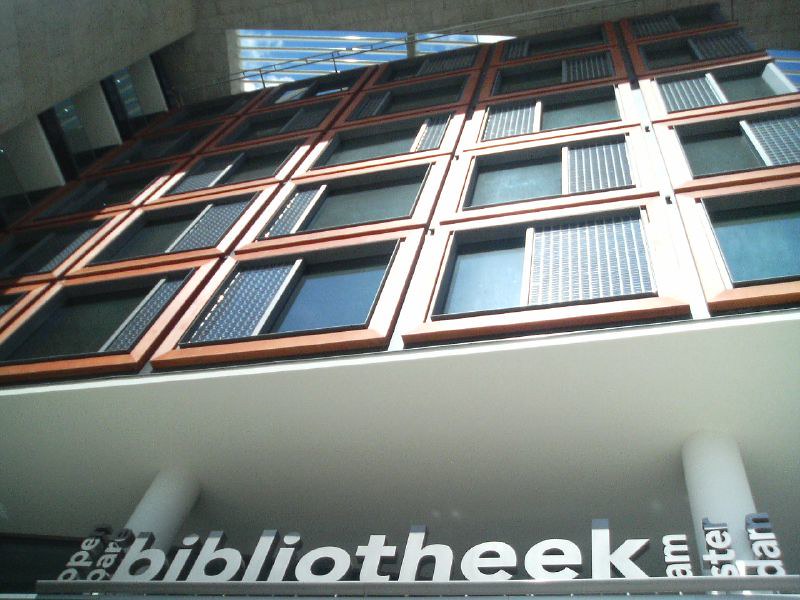The photograph captures a striking, upward-angled view of a distinctive building. At the base, prominently displayed in silver-painted, standalone letters, is a sign reading "Open Bear Bibliotheque." This sign is supported by two prominent white beams that accentuate the building’s modern design. The façade features multiple windows framed in orange, giving a lively and contemporary feel. Above these windows, skylights reveal a clear blue sky, enhancing the sense of openness. The building appears almost free-floating due to its unique architectural style and seems designed more for aesthetic appeal than for practical entry by people.